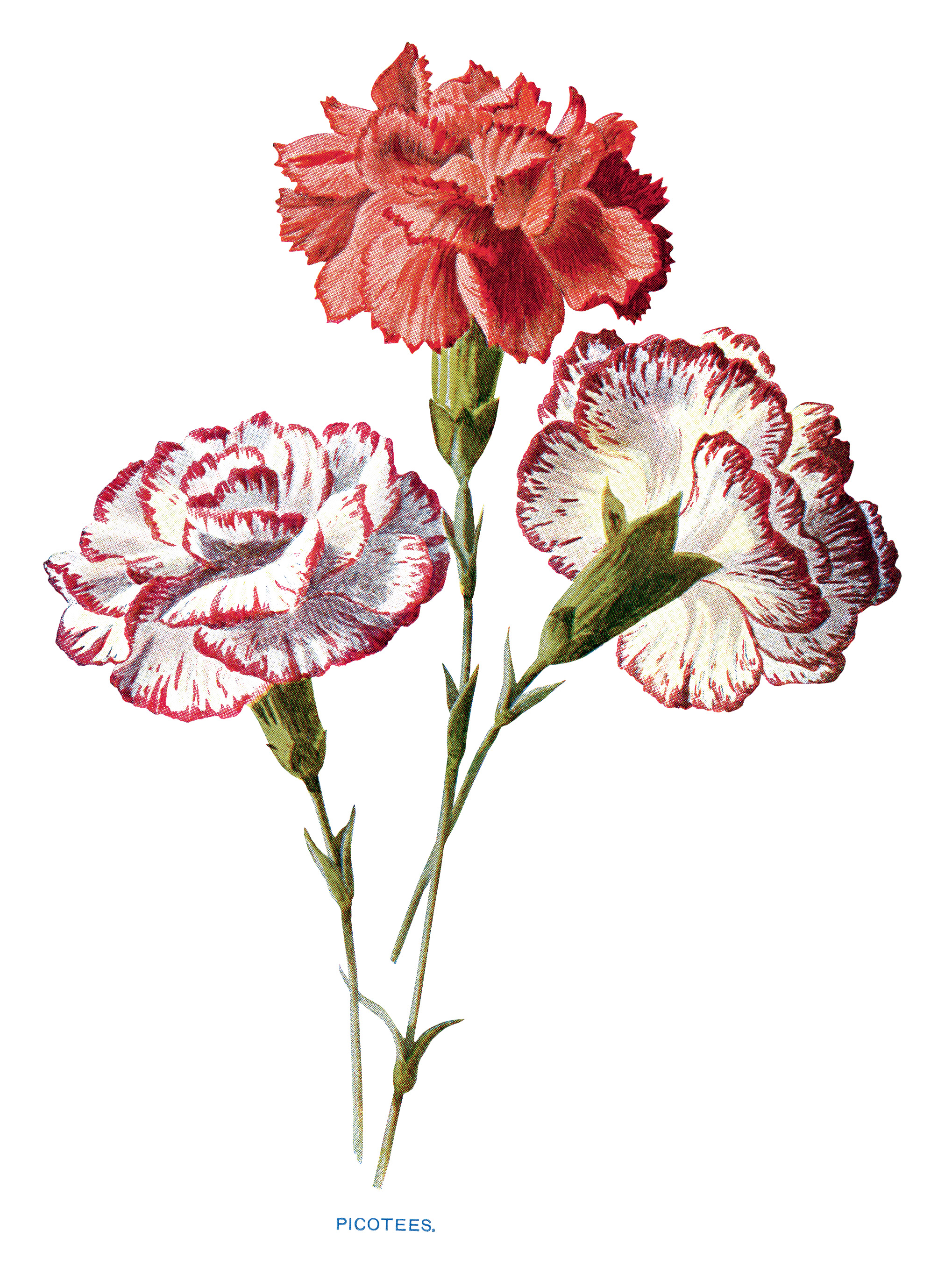This is a detailed illustration of three flowers against a white background, labeled "Picotes" in blue lettering at the bottom. The composition features three long-stemmed flowers, identified as carnations. The middle flower stands tallest with a green stem and boasts solid red petals, which are darker at the edges. Flanking this central bloom, the flowers on the left and right have slightly shorter, green stems and are white with pinkish-reddish trims around their petals. The flower on the right appears to be angled away, showing primarily the back of its white petals edged in dark pink. Each flower has three distinct layers of petals, adding to the intricate detailing of the illustration.